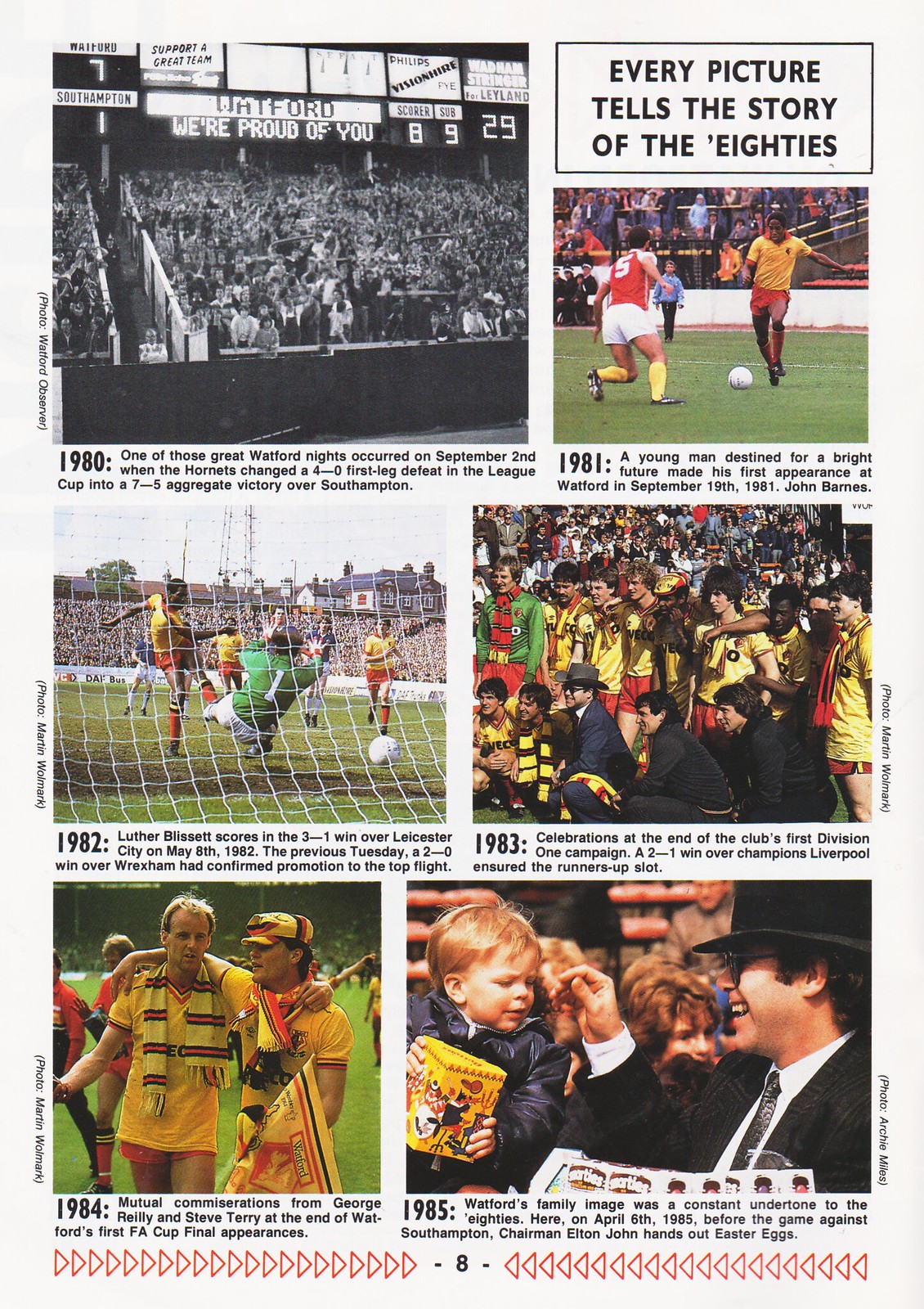The image is a magazine page showcasing a visual history of a soccer club through the 1980s, featuring six photographs arranged in a 2x3 grid. The top section features two photographs: the left one, a black-and-white image from 1980, shows enthusiastic fans in the stands with a sign reading "Watford, we're proud of you," and a scoreboard displaying scores like 8-9 and 7-1. The right photograph, dated 1981, is somewhat blurred but reveals players on a grassy field with a crowd in the distance and the caption "every picture tells a story of the 80s."

The middle row presents a diverse scene of soccer activities: the left photograph from 1982 captures the moment a player shoots past the goalie towards scoring; the right, dated 1983, shows a group of players possibly celebrating or preparing for a game with an audience in the background.

In the bottom row, the left image from 1984 features two soccer players in yellow jerseys holding a flag on the field. The final picture, marked 1985, shows a touching moment between a man in a black suit and top hat caressing a young boy's hair, with the boy holding a box, possibly of food. Both stand on the grassy field with the audience barely visible in the background. A caption above all images reads, “Every picture tells the story of the 80s,” tying together this nostalgic visual journey.